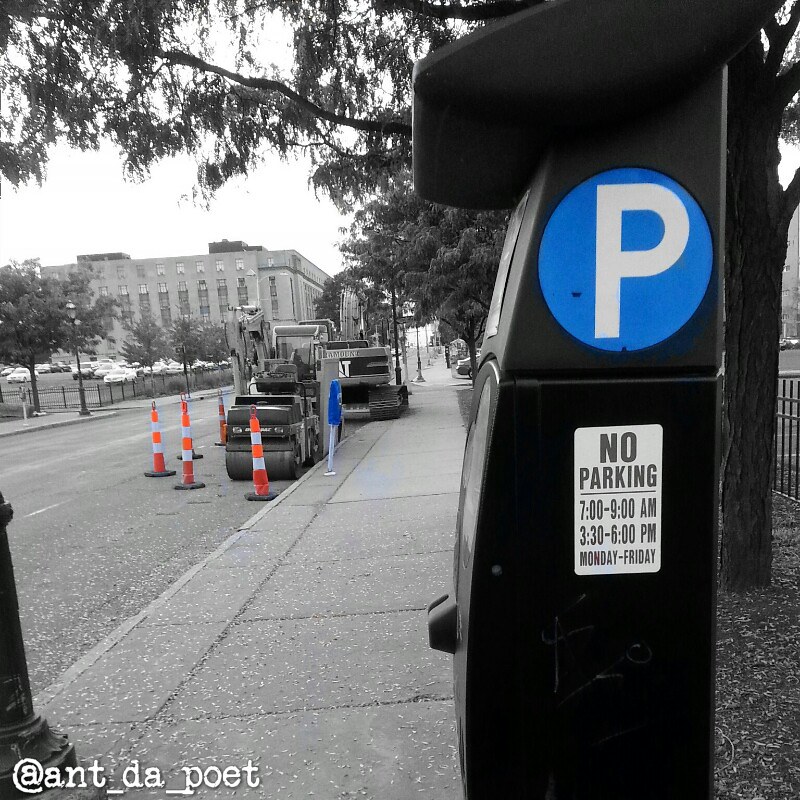The image captures a city street scene characterized by a mix of black and white with selective color accents in orange and blue. On the right-hand side, a sidewalk stretches alongside a multi-level building and a parking lot filled with cars. Trees line both sides of the street, enhancing the urban landscape. Prominently, there are construction machines, including a steamroller and an excavator, surrounded by orange and white striped cones. A notable element is the parking meter kiosk, displaying blue coloring with a white "P" and a sign indicating restricted parking times (7 to 9 a.m., 3:30 to 6 p.m., Monday through Friday). The image composition focuses on the activities and features in front of the multi-story building in the background, emphasizing the blend of construction and urban details.